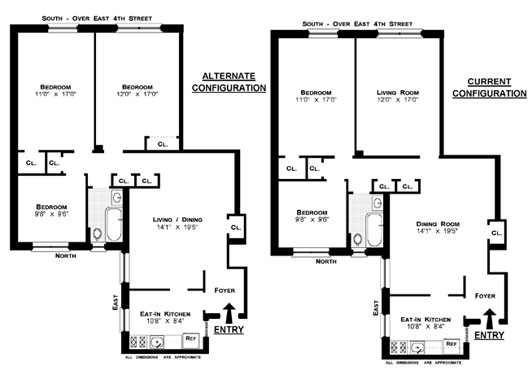The image showcases two side-by-side, black-and-white blueprints labeled "Alternate Configuration" and "Current Configuration." Both blueprints are titled "South Over East 4th Street" at the top. Each blueprint details a layout featuring three different bedrooms with specific dimensions. 

In the "Alternate Configuration" on the left:
- The first bedroom is 11'0" x 17'0".
- The second bedroom measures 12'0" x 17'0".
- The bottom-left bedroom has dimensions of 9'8" x 9'8".

In the "Current Configuration" on the right:
- The dimensions remain consistent with the "Alternate Configuration."

Other shared features in both layouts include:
- A living room adjacent to the bottom bedroom, measuring 14'1" x 19'5".
- A foyer located below the living room with an entry point clearly marked by an arrow.
- An eat-in kitchen at the bottom of the layout, measuring 10'8" x 8'4". 

Overall, the detailed black-and-white blueprints offer a comprehensive overview of the space arrangements in both proposed configurations.